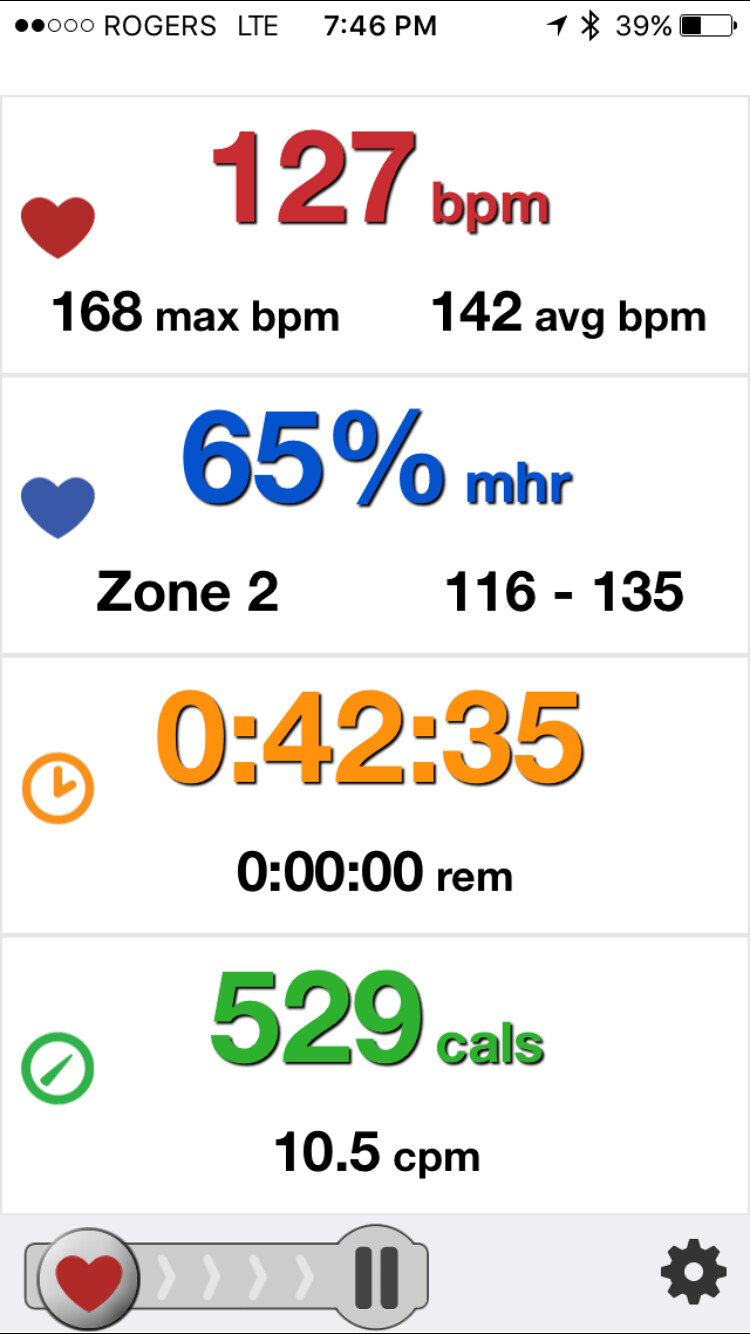The screenshot is from a health tracking app displayed on a cell phone at 7:46 PM, with the battery at 39%. The app shows detailed health statistics: a heart rate of 127 BPM in red, a maximum BPM of 168, and an average BPM of 142. The user's current effort is 65% of their maximum heart rate (MHR), placing them in "Zone 2" which ranges from 116 to 135 BPM. A clock icon indicates a session time of 42 minutes and 35 seconds, and there's an entry showing 529 calories burned. Notably, the app also highlights statistics like 10.5 CPM (likely steps or movements per minute). The interface includes various icons such as a heart on a meter, a settings gear, and a blue heart next to the MHR. The phone has a low signal with only two out of five bars filled and is connected via Rogers LTE.